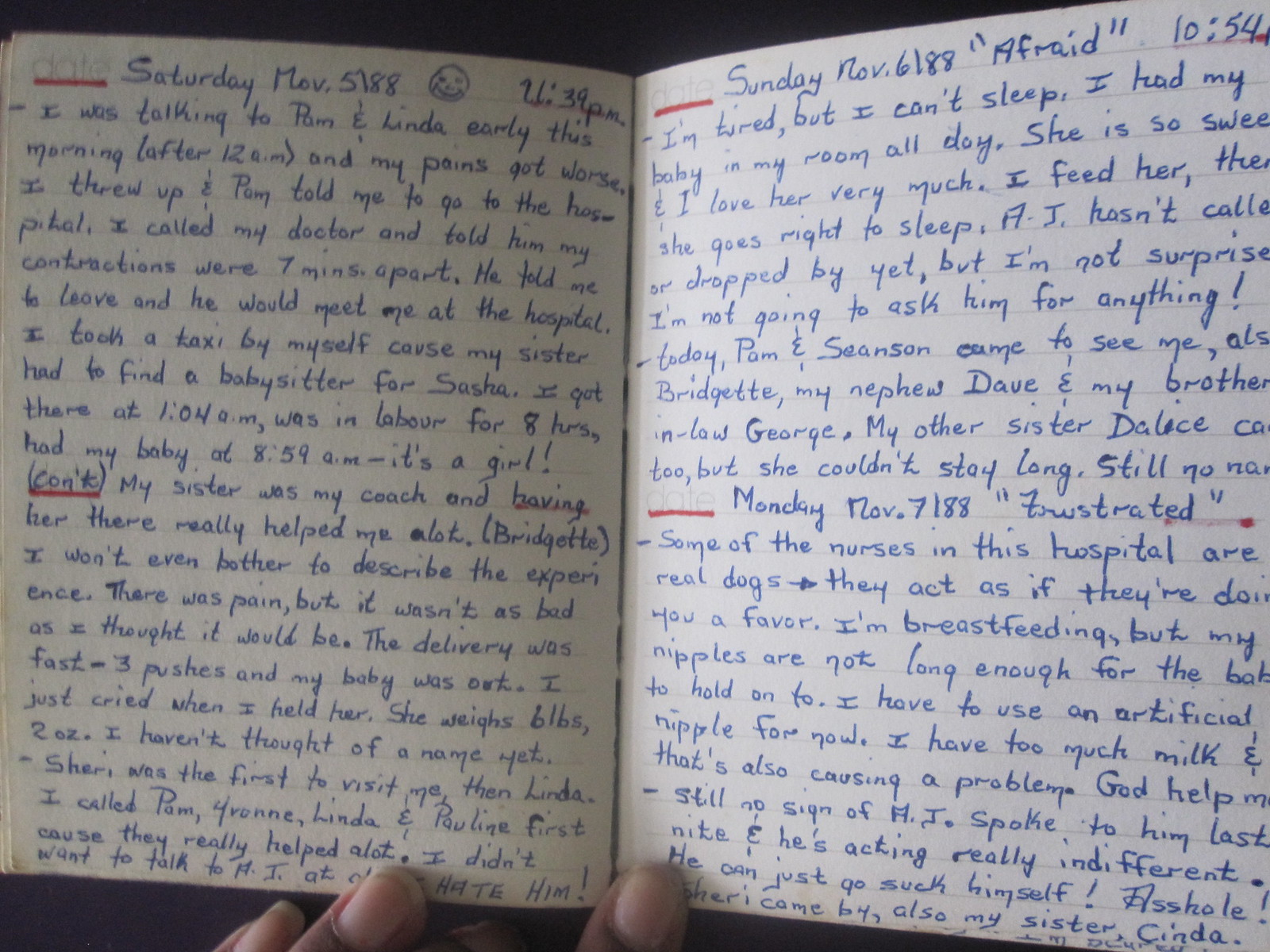The photograph depicts an open diary, revealing two handwritten pages in blue ink on white-lined paper. The left page is dated "Saturday, November 5, 1988" at 11:39 p.m., featuring a smiley face and chronicling a woman's journey through labor. She describes late-night conversations with Pam and Linda, increasing contractions, and vomiting before heading to the hospital alone in a taxi due to her sister's need to find a babysitter for Sasha. She arrived at 1:04 a.m., endured an eight-hour labor, and gave birth to a baby girl at 8:59 a.m. Her sister and coach, Bridget, provided significant support during the delivery, which took only three pushes. The entry notes the baby's weight as six pounds, two ounces, and details visitors including Sherry, Linda, Pam, Yvonne, and Pauline. Notably, she expresses disdain for a person abbreviated as "AJ."

The right page, underlined in red, reads "Sunday, November 6, 1988," and is titled "Afraid" at 10:54 (a.m. or p.m. not specified). The new mother writes about her exhaustion yet inability to sleep, her baby's sweetness, and relief that AJ has not contacted her. Visitors that day included Pam, Shonson, Bridget, her nephew Dave, her brother-in-law George, and her sister Delise, who couldn’t stay long. Still unresolved is the baby's name.

A red underline marks the beginning of the next entry: "Monday, November 7, 1988," titled "Frustrated." She vents about the unkind hospital nurses and troubles with breastfeeding due to short nipples and excess milk. She reflects on AJ’s indifferent behavior, expressing anger towards him, and mentions visits by Sherry and her sister Cinda. Throughout, the diarist's emotions vividly convey the realities of her childbirth and early motherhood experience.